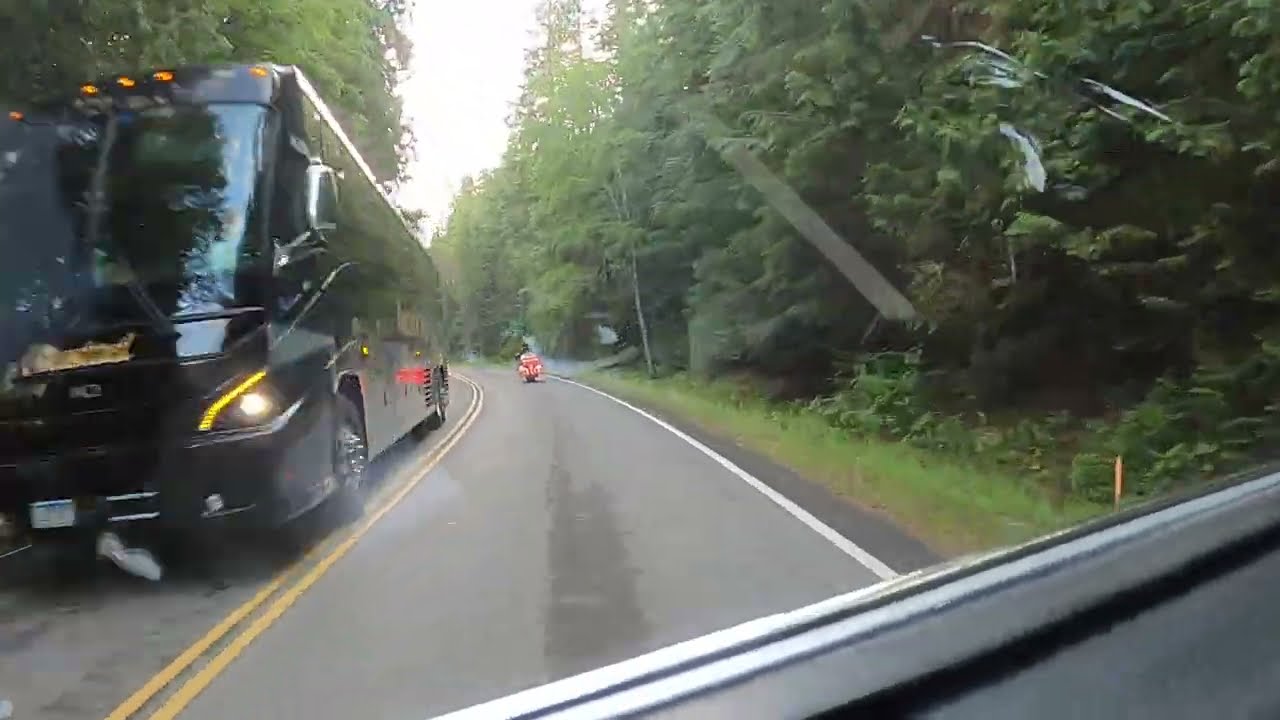The image, taken from the inside of a vehicle possibly via a dash cam behind the windshield, depicts a two-lane road with double yellow dividing lines indicating no passing is allowed. The road appears slightly wet, suggesting recent rainfall, with a couple of streaks on the windshield adding to this impression. The vehicle is positioned on the right side of the road, and up ahead in its lane is a red motorcycle or scooter. On the opposite lane, a black bus with red stripes and a precariously hanging white piece of paper is traveling in the opposite direction, quite close to the center line. Both sides of the road are lined with tall, thick trees and there is a grassy ditch on the right. The sky is glaringly white, contributing to the overall bright yet overcast atmosphere of the scene.